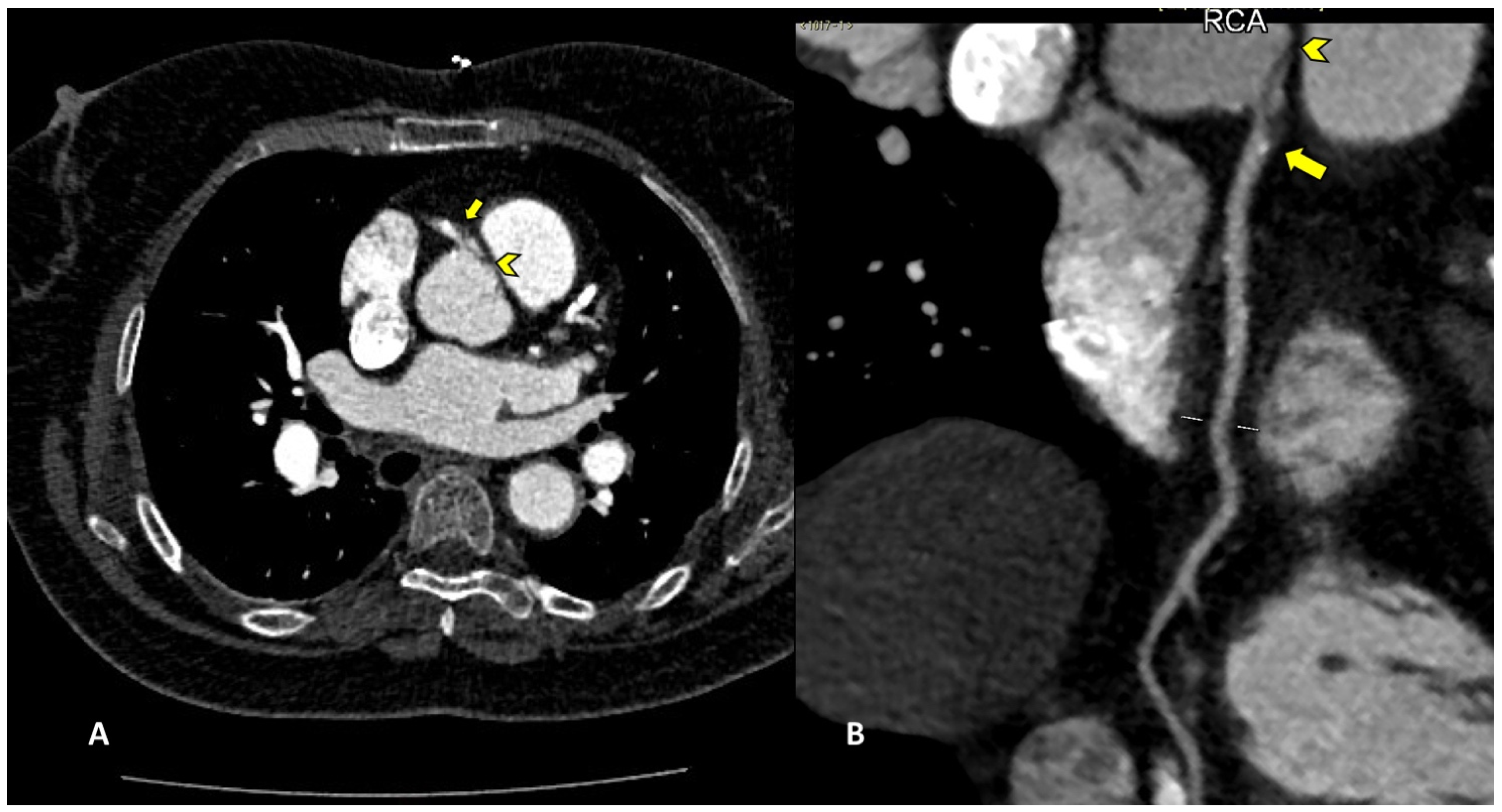This detailed, horizontally oriented photograph appears to be an MRI scan, displaying a black background with various shades of gray to indicate internal structures. Detailing a cross-section of what seems to be a human torso, the image splits into two main panes: the left side labeled 'A,' showing a broader view of the torso, and the right side labeled 'B,' offering a close-up of specific areas. Each pane features both standard yellow arrows and chevron arrows, pointing to areas of interest. The arrows are strategically placed, with one specific cluster focusing on some irregularly shaped white objects that could be indicative of pathological conditions, such as cancer cells. At the top right corner, the letters 'RCA' are prominently displayed in a white font. Overall, the photograph also includes some circular structures and what might be a vein, hinting at a complex and nuanced internal landscape. The photo appears to have been computer-enhanced, with superimposed yellow arrows guiding the viewer's attention to critical areas within this diagnostic image.